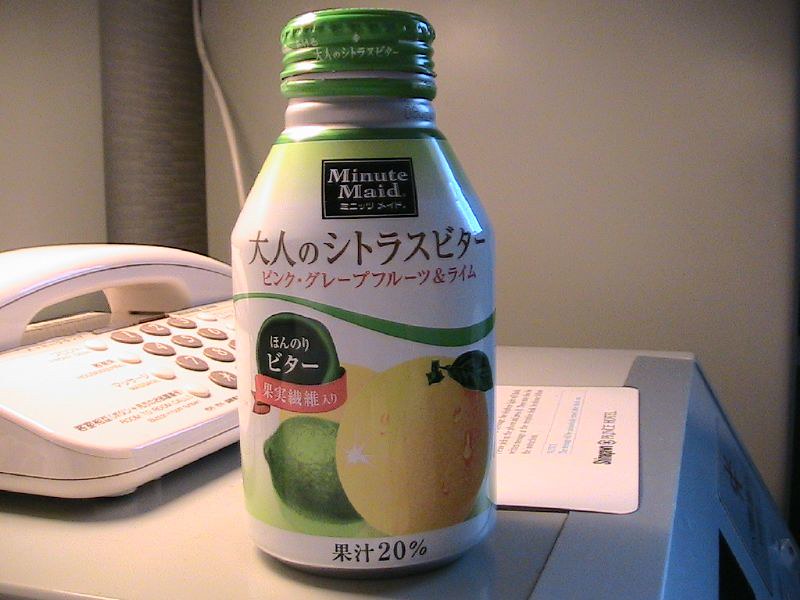This photograph showcases a bottle of juice produced by Minute Maid. The label, adorned with Chinese or Japanese lettering, prominently features illustrations of oranges and limes, possibly lemons and limes, indicating the flavor profile of the beverage. At the bottom of the label, "20%" is displayed, suggesting that the juice content is 20%. The bottle, constructed from metal or aluminum, has a distinctive green cap and is open. It is positioned on a countertop or desk, with a telephone visible behind it and a sheet of paper situated to the right.